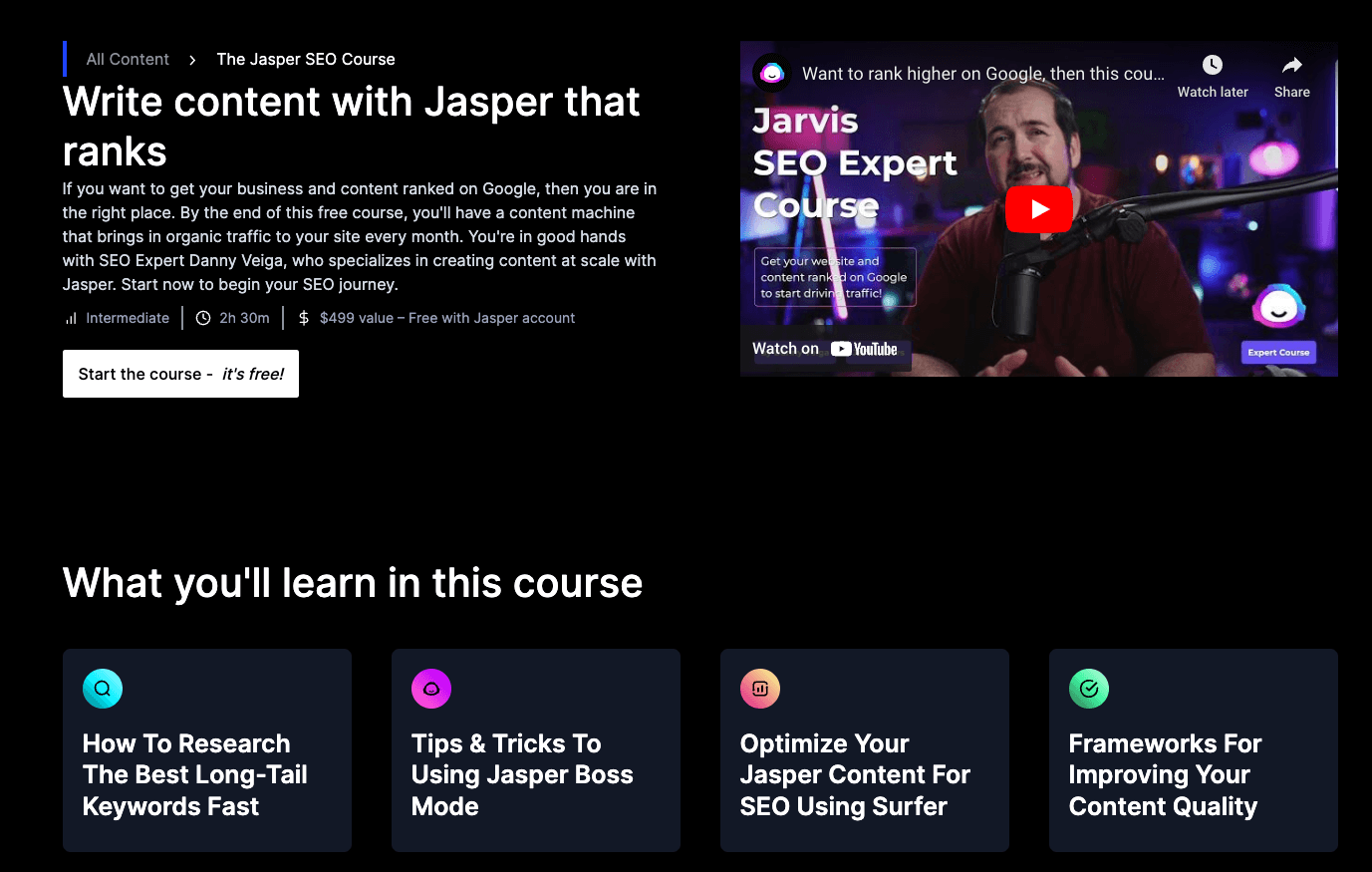This image depicts a screenshot of a web page set against a solid black background. At the bottom part of the image, there are four colored circles, each featuring a distinctive icon and accompanied by descriptive text. From left to right:

1. A small blue circle with a magnifying glass icon. Below it, in bold white text, is the title: **"How to Research the Best Long Tail Keywords Fast."**
2. A purple circle with an icon representing tips and tricks. This is followed by the text: **"Tips and Tricks to Using Jasper Boss Mode."**
3. An orange and pink circle next in line, which has an icon for optimization, accompanied by the text: **"Optimize Your Jasper Content for SEO Using Surfer."**
4. Lastly, a green circle with a black checkmark icon, followed by the text: **"Frameworks for Improving Your Content Quality."**

In the upper right corner of the image, there is a video thumbnail with the YouTube icon centered. The video title displayed is: **"Jarvis SEO Expert Course."**